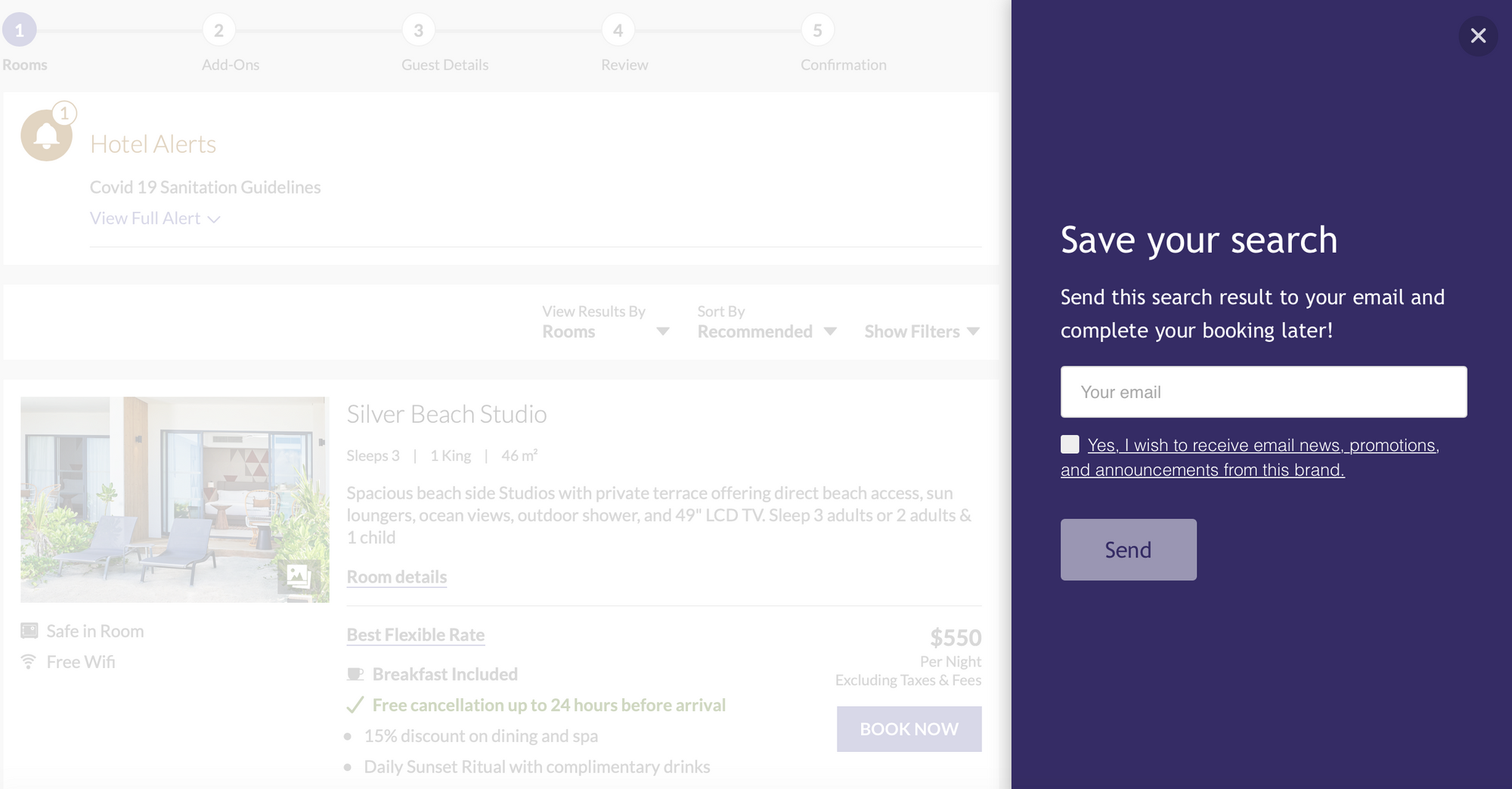The website image presents a user interface for booking a hotel stay. The left-hand side of the image is faint and very light gray. At the top of the page, a navigation bar guides the user through five steps: "1. Rooms," "2. Add-ons," "3. Guest Details," "4. Review," and "5. Confirmation." Below this navigation bar, a circular icon featuring a bell is labeled "Hotel Alerts," with a subtext mentioning "COVID-19 Sanitation Guidelines" and a link to "View Full Alert."

Further down, the interface displays various columns with actionable items: "View Room," "View Results by Room," "Sort by Recommended," and "Show Filters.” On the left side, there is a photo of what appears to be a hotel lobby, adorned with chairs, plants, and blue walls in the background. To the right of this photo, text identifies the room as "Silver Beach Studio."

Positioned further to the right is a dark blue text box. In the upper right-hand corner of this box is a white "X" for closing it. Central to the text box is a field labeled "Your Email," where users can input their email addresses. Beneath this field is a checkbox with a sentence stating, "Yes, I wish to receive email news, promotions, and announcements from this brand." At the bottom of the text box is a gray button labeled "Send."